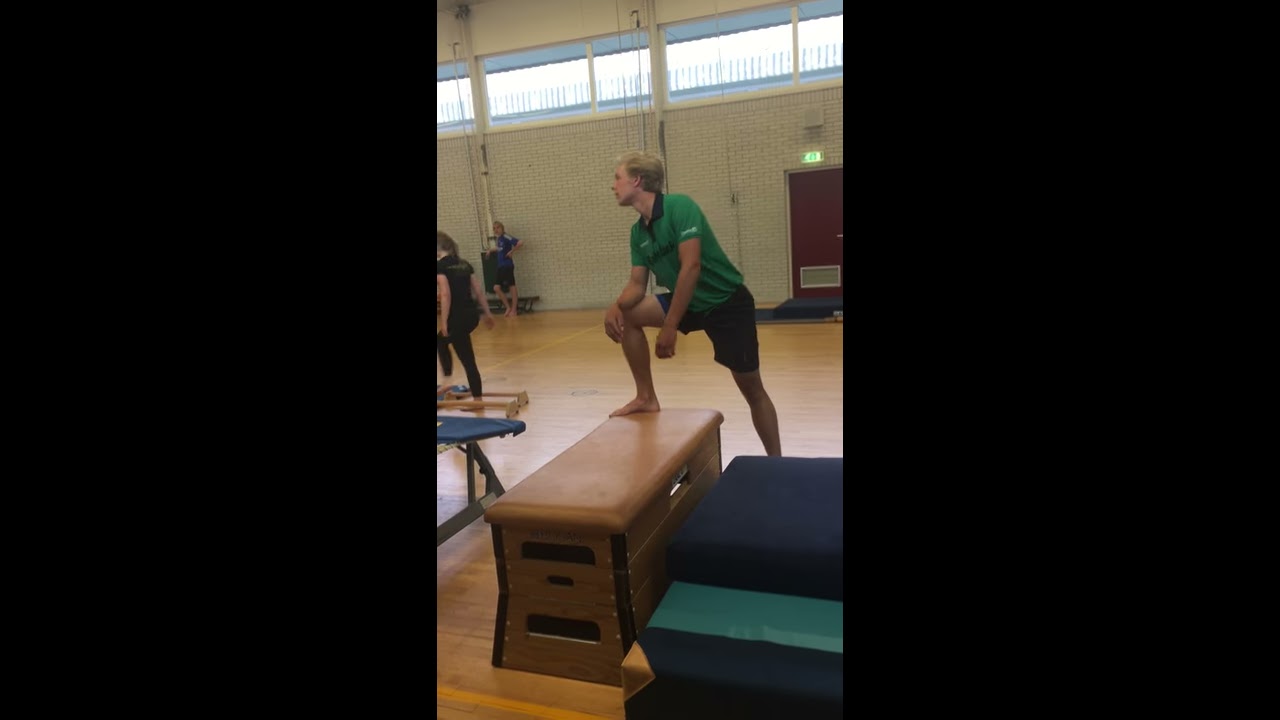In this detailed image from inside a gymnasium, a young man wearing a green shirt with a black collar, paired with black shorts, is prominent in the foreground. He is positioned on a brown gymnastic vaulting horse, which appears to be a padded rectangular structure with handle holds and brown padding on top. His left knee is bent and resting on the vaulting horse, while his right leg is fully extended. His elbow is bent, and his hand rests on his knee. The young man, a white male with short blonde hair, faces slightly towards the left while his body is directed forward, looking towards the camera.

Adjacent to the vaulting horse are two blue steps, each featuring lighter and darker blue stripes, aiding in mounting the equipment. The gymnasium itself has a light tan wooden floor and high white brick walls. Elevated windows allow natural light to shine through, giving the space an airy feel. In the background, another person wearing a black shirt and black pants can be seen exercising, while a young woman in black leotards appears further to the left of the image. A red door with an exit sign above it is situated on the right-hand side, adding to the gym's typical layout. The overall scene suggests an active environment, possibly a gymnastics or fitness class, captured with the intimate frame of a smartphone image.